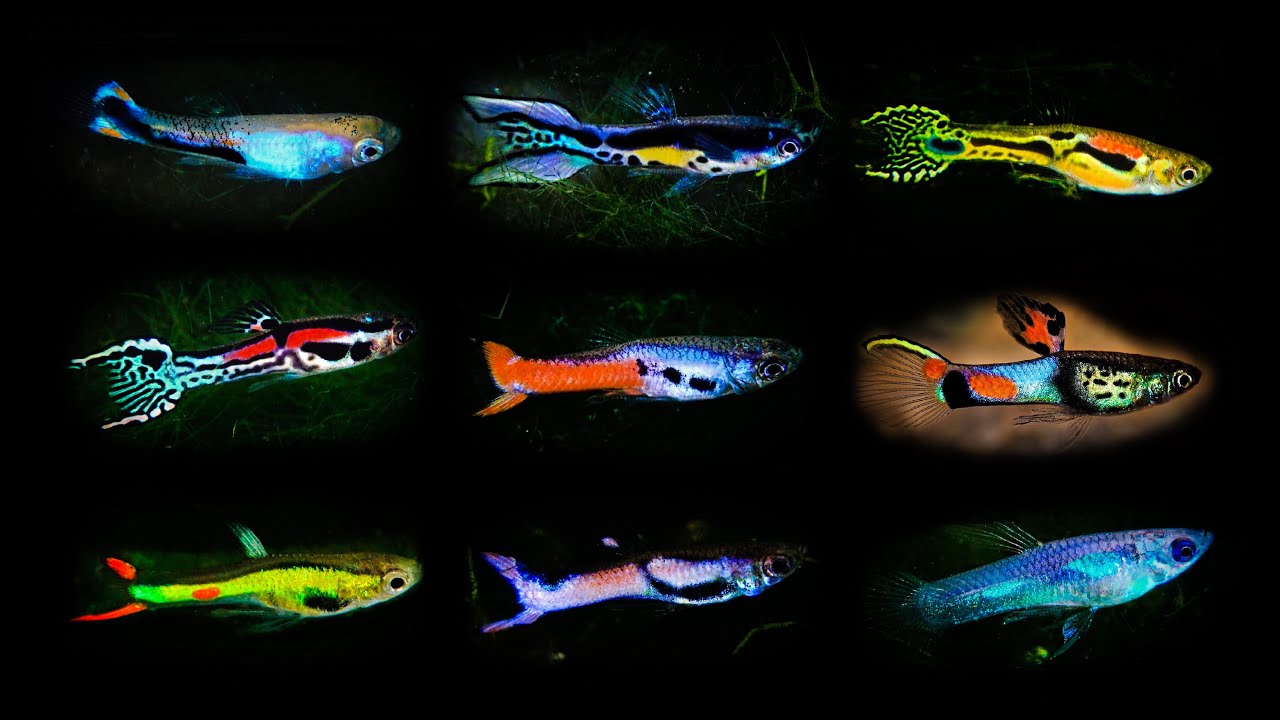The image showcases a vibrant collage of nine distinct and colorful fish arranged in a 3x3 grid format against a vivid black background, enhancing the striking hues of the fish. These small tropical fish, possibly tetras or guppies, display an array of dazzling colors including bright blues, yellows, reds, oranges, and greens, making each one uniquely eye-catching. The fish vary from predominantly single colors to multicolored patterns; some have clear fins or black accents, while others display elaborate tails that fan out like a bell or fork. Each fish swims left to right, with features such as blue bodies with dark blue eyes, red and yellow combinations, and even prehistoric-looking forms adding to the visual interest. This playful and detailed arrangement against the black background creates a vivid contrast that celebrates the neon vibrancy of the fish's colors.